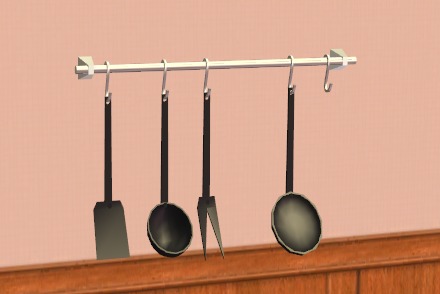This detailed image showcases a peach-colored wall with a wooden wainscoting below it, featuring a decorative horizontal bar. The wainscoting, a light brown hardwood with an added decorative strip, provides a charming rustic accent to the scene. Hanging on the wall is a silver metal rod rack equipped with S hooks, from which several matte black kitchen utensils dangle. From left to right, these utensils include a large flat spatula, a sizable ladle, a two-pronged fork, and another ladle, slightly larger than the first. One S hook on the right end remains empty. Notably, the rod, hooks, and overall composition possess an illustrative, almost cartoon-like quality, adding a distinct character to the photo.